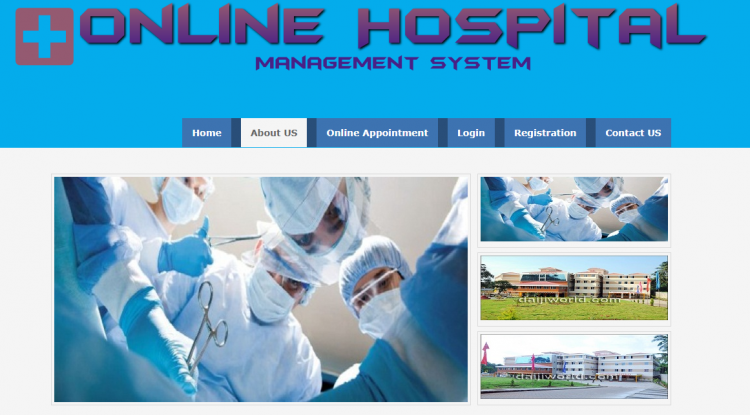This image showcases the homepage of an online hospital management system. At the top of the interface, there are navigational links including "Home," "About Us," "Online Appointment," "Login," "Registration," and "Contact Us." The background features buildings with a prominent watermark that reads "daijubo.com." In the foreground, several doctors and nurses are visible, appearing to perform a medical operation, emphasizing the healthcare services promoted by the website.